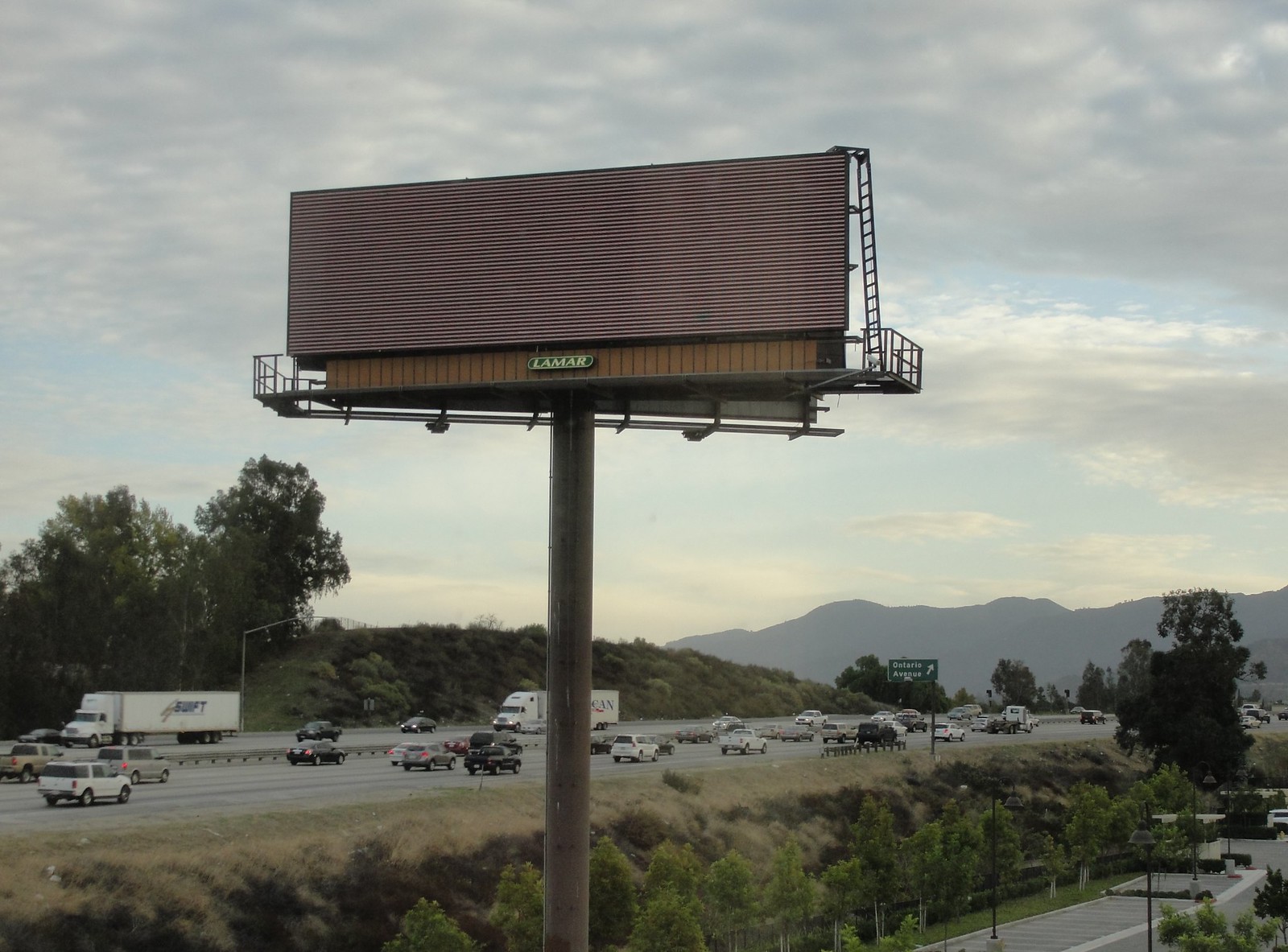In this image, the focal point is a weathered and rusted, dark brown metal billboard supported by a well-rusted pole. The billboard is devoid of any advertisements, with a noticeable logo "Lamar" displayed below on a brown or black plaque. Adjacent to the billboard, a ladder is fixed on the right side. The scene is set along a busy highway, with more vehicles populating the side heading into the distance. In contrast, the side of the highway heading towards the left of the image has notably fewer vehicles and includes two semi-trucks. The highway itself is elevated, and there's a grassy downhill slope leading to a lower segment of the road. The backdrop includes lush green hills and numerous trees, with distant mountains adding depth to the scene. The sky is clear with white clouds, and despite the detailed landscape, the lighting suggests that the photo might have been taken during an overcast, possibly dusk, time of day.